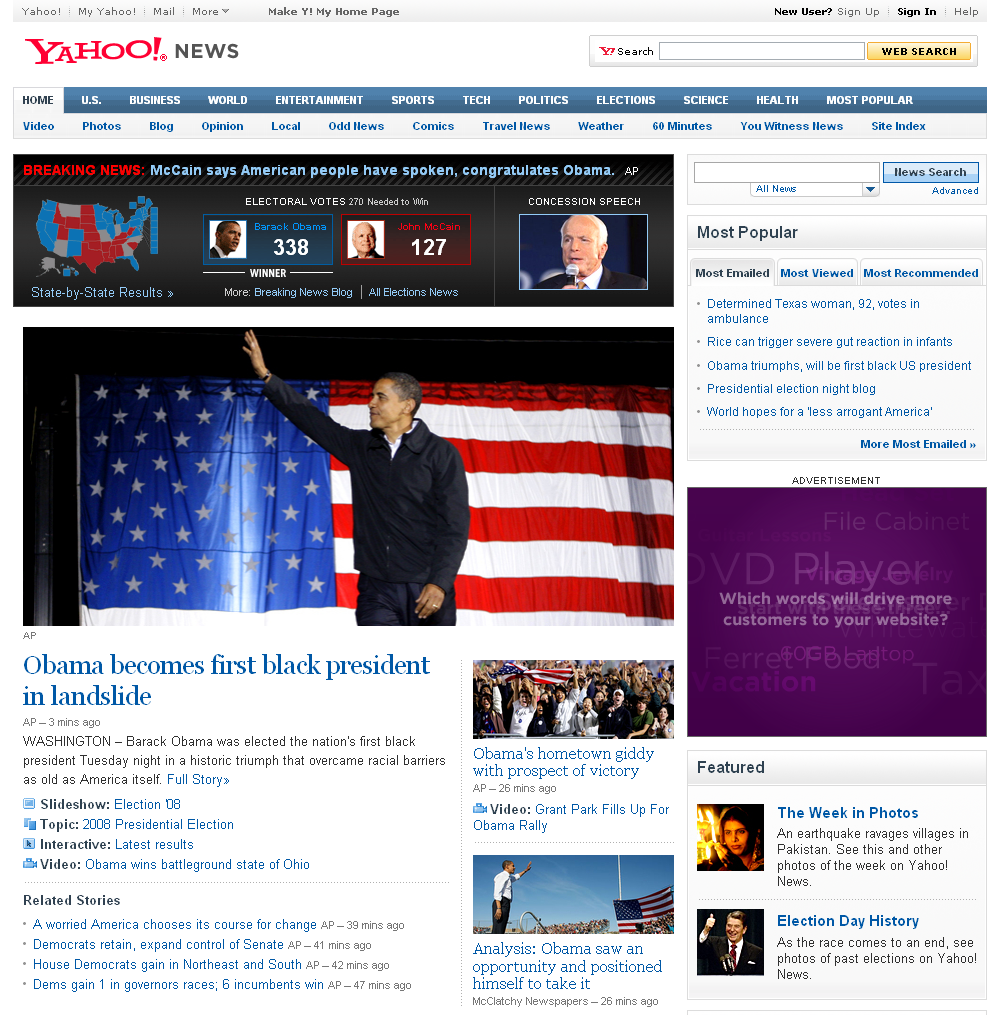The image showcases a Yahoo News webpage, prominently featuring election coverage. In the upper left corner, options for Yahoo, MyYahoo, Mail, and More are visible, while the upper right corner displays options for New User Sign Up, Sign In, and Help. The Yahoo! logo is prominently displayed in red, followed by "News" in black. A search bar with a yellow search button is also situated in the upper right corner.

The navigation bar at the top lists several categories: Home, U.S., Business, World, Entertainment, Sports, Tech, Politics, Elections, Science, Health, and Most Popular. The Home category is selected, revealing a drop-down menu with additional options like Video, Photos, Blog, Opinion, Local, Odd News, Comics, Travel, Weather, 60 Minutes, Your Witness News, and Site Index.

The main section is headlined by "Breaking News," featuring electoral results and updates. The highlighted headline states, "McCain says American people have spoken, congratulations Obama," with detailed election coverage including state-by-state results, Breaking News Blog, and All Election News. Electoral votes are shown with Barack Obama at 338 and John McCain at 127, announcing Obama's historic victory as the first black president of the United States.

The page also includes sections titled "This Week in Photos" and "Election Day History." In the upper right corner, articles are highlighted under various headlines such as "Determined Texas Woman, 92, Votes in Ambulance," "Rice Can Trigger Severe Gut Reaction in Infants," "Obama Triumphs, Will Be First Black President," "Presidential Election Night Blog," and "World Hopes for Less Arrogant America." The content captures the significant triumph of Barack Obama breaking racial barriers and the global anticipation for a transformative American leadership.